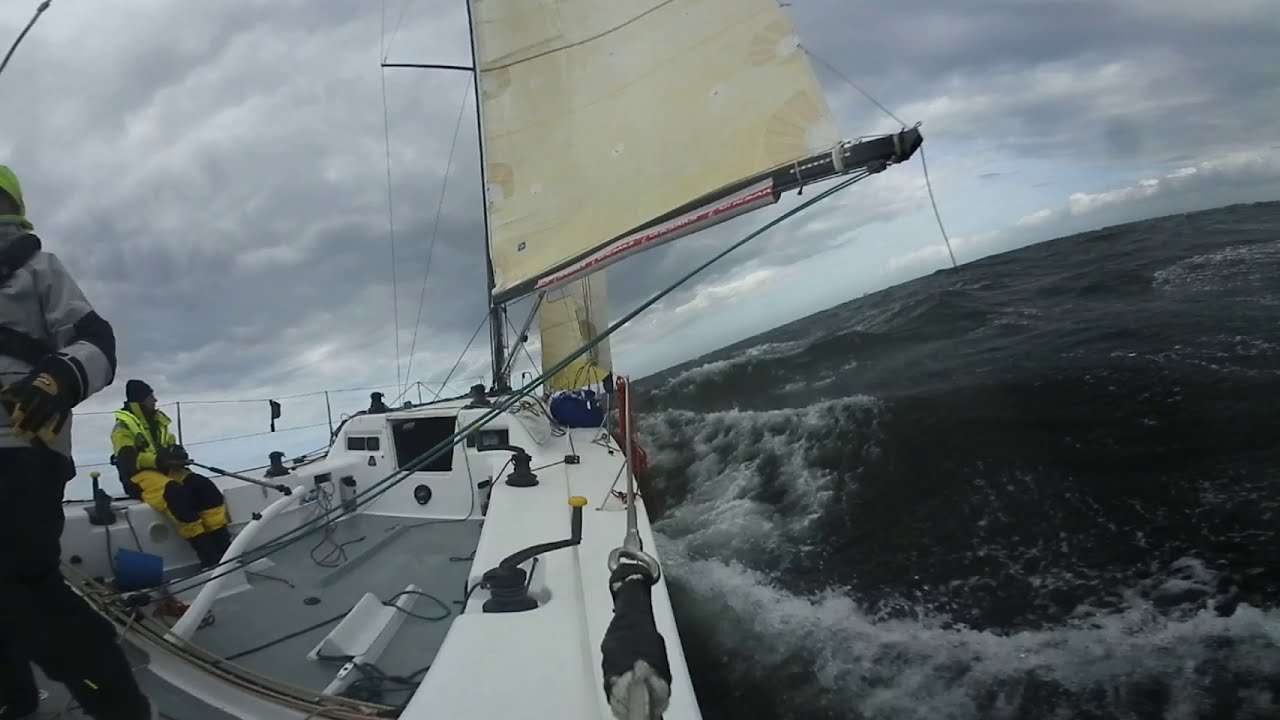The image captures a turbulent scene of a sailing boat navigating through rough, choppy waters under a largely gray sky filled with storm clouds, with some blue peeking through around the horizon. The sea appears greenish, with white crests on the waves indicating the rough conditions. Central to the image is a white sailing boat equipped with white sails and a black sail bottom. It is further highlighted by various visible details such as black fishing rods, a blue bucket, and a blue bag positioned on the deck.

Onboard, there are two people braving the harsh weather. One person is standing to the left of the camera wearing waterproof clothing, including a reflective beanie or yellow hat and a gray and black coat complemented by black pants. The second person is seated on the left side of the boat, dressed in a yellow outfit with black knee pads, arm pads, and black boots, and is wearing a black beanie hat. This person appears to be handling a pole, likely the boat's tiller.

The boat's deck is gray and cluttered with various sailing tools and wiring, contributing to a sense of activity and readiness amidst the stormy sea. The wide-angle and fish-eye perspective of the image, likely taken from an action camera like a GoPro, emphasizes the dynamic and expansive nature of the scene, capturing both the threatening sky and the turbulent waters.